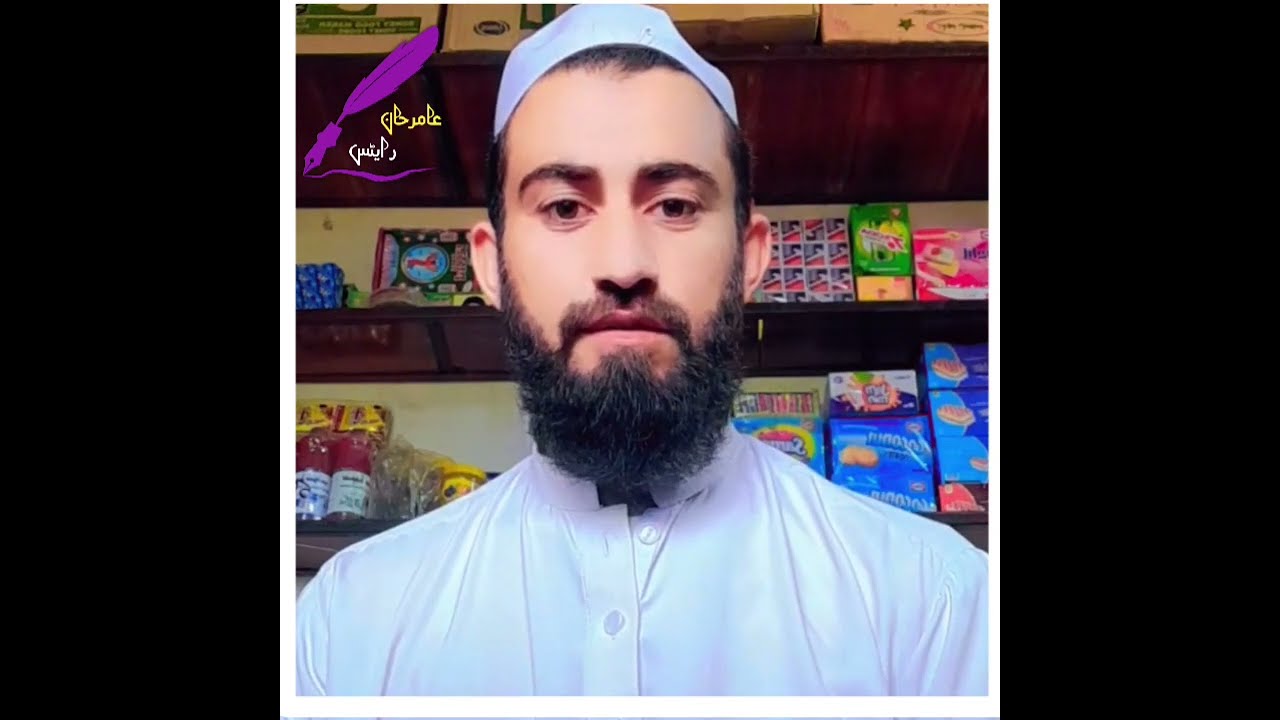The photograph features a young Arabic man running a grocery store, centrally framed within a square image bordered by a white frame. The background reveals a variety of colorful packages that resemble food, candy, or possibly fireworks, neatly arranged on wooden shelves. The man, dressed in traditional Muslim attire, sports a light blue buttoned-up shirt and a matching religious headgear resembling a yarmulke. Notably, his beard is short and curly. Above the packages, there are cardboard boxes on the top shelf, and in the upper left corner, an icon and some Arabic text are visible. The man's expression is neutral as he looks directly at the camera, suggesting the photo might have been taken with a webcam. The entire visual is set against two black bars on each side, filling the remaining space within the high-definition TV-shaped image.